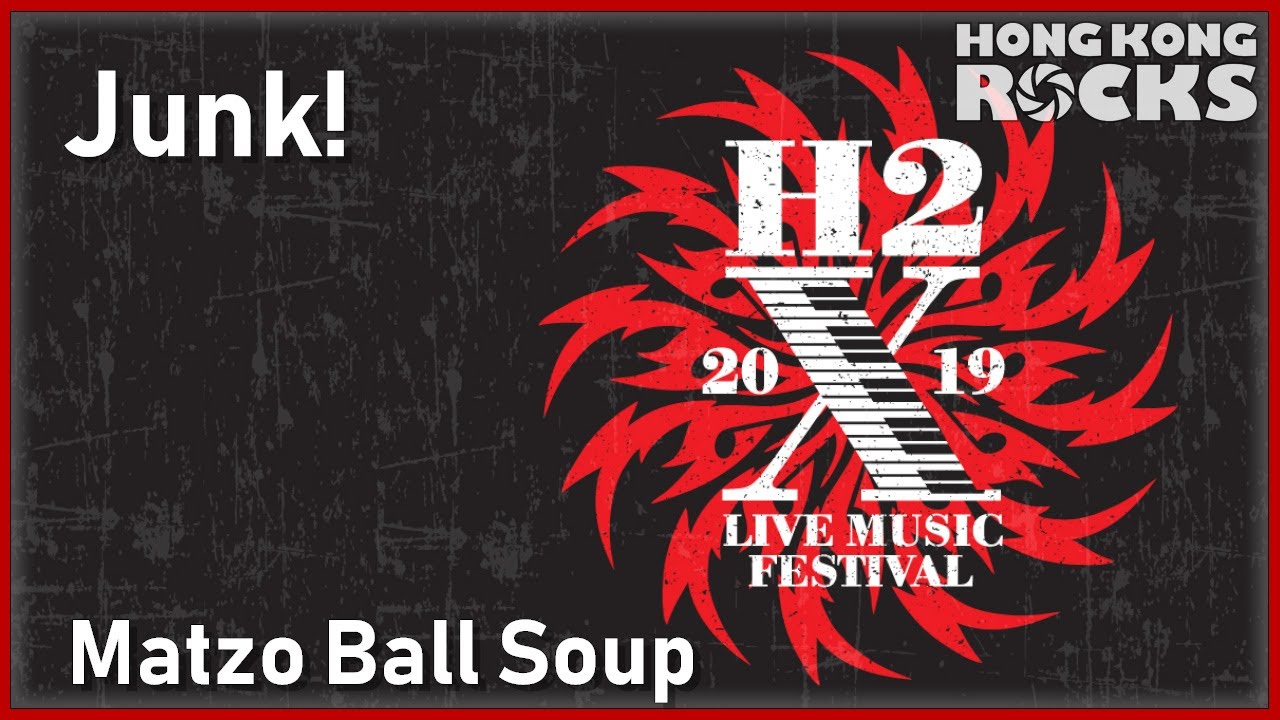This poster is for a live music festival that took place in the second half of 2019. The image is horizontally oriented and primarily features a black background with subtle grey streaks. A stylized red spiral design, reminiscent of a buzzsaw, takes up about 40% of the right side of the image. Superimposed on this red spiral are the letters H and the number 2 along with a keyboard. The characters "20" are on one side of the H2, while "19" is on the other, together forming "2019." Below this design, the text "Live Music Festival" is prominently displayed.

In the top right corner, in all capital letters and a pale grey font, the phrase "Hong Kong Rocks" appears, with the letter "O" mimicking the red spiral design. On the top left corner, the word "Junk!" is written, likely indicating a band name. The bottom left corner features the text "Matzo Ball Soup" in bold, white letters, suggesting it is another band's name. The image's color palette is restricted to black, white, and red, creating a visually striking advertisement for the festival.